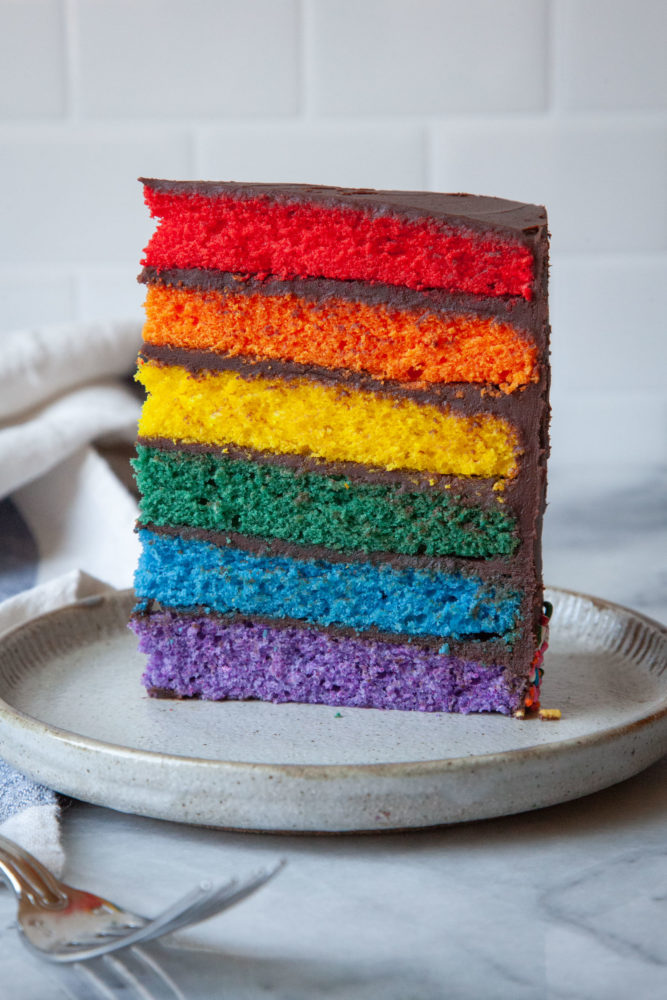This vibrant color photograph showcases an eye-catching slice of rainbow cake, displayed on a light blue ceramic plate adorned with brown speckles. The cake features six distinct layers, each boasting a vivid hue: bright red, bright orange, bright yellow, bright green, bright blue, and bright purple. Between each of these colorful layers is a generous spread of rich chocolate frosting. The cake is topped with a glossy black frosting, adding a touch of elegance. The plate rests on a pristine white marble surface with striking black veins, accompanied by the tines of a silver fork on the right. To the left of the plate, a green and white napkin is partially visible, along with another piece of folded white fabric. The backdrop of the image is a white-painted brick wall, providing a simple yet stylish contrast to the vivid colors of the cake.